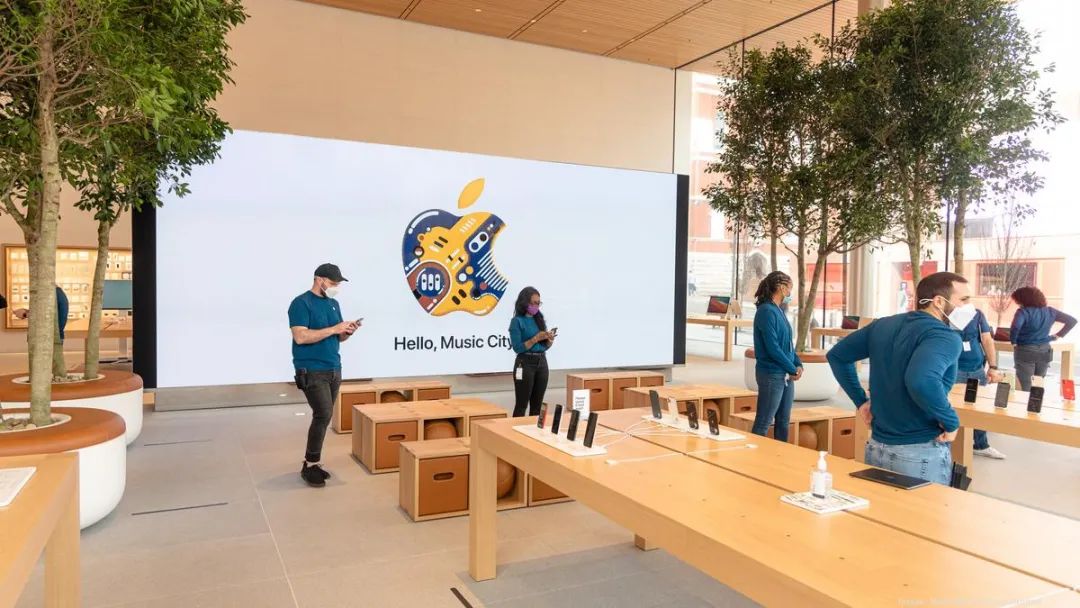This color photograph captures the spacious interior of what is unmistakably an Apple Store, designed with earthy, brown tones that exude a warm and inviting atmosphere. The store's decor prominently features natural elements, with two large, circular white plant pots, each topped with wood and housing tall trees, situated on both the left and the right sides of the image. These planters and trees are symmetrically placed, enhancing the store's organic and modern aesthetic.

The left side of the store boasts tall windows that flood the space with abundant natural light, creating a vibrant environment. The back wall, which is painted brown, prominently displays a large white banner bearing the iconic Apple logo. This banner features a vivid design mainly composed of blue and yellow colors, with touches of red and white, and the welcoming phrase "Hello Music City" written beneath it.

The store is bustling with activity, as numerous Apple employees, identifiable by their uniform dark blue shirts, are scattered throughout the space. These shirts vary between long sleeves and short sleeves, paired with blue jeans or gray pants. The employees are all adhering to health guidelines by wearing face masks, which vary in appearance from plain white to patterned designs.

Wooden tables are strategically arrayed starting from the bottom right corner of the image, showcasing a variety of iPhones on display. Additionally, a bottle of hand sanitizer is placed on one of the tables, underscoring the store’s commitment to cleanliness and safety. The photograph is wider than it is tall, capturing a broader view of the well-designed, contemporary interior of this Apple Store in Music City.